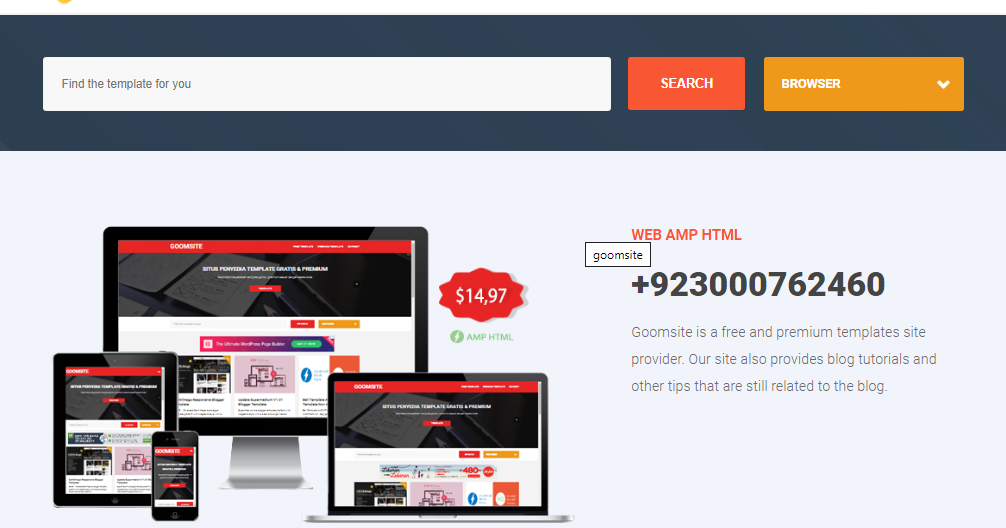This is a cropped screenshot of a website. The top section features a dark gray header. On the left side of this header, there is a white rectangular search bar with the small, medium gray placeholder text that reads, "Find the template for you." To the right of the search bar, a red button labeled "SEARCH" in all caps, and an elongated orange button with white text on the left that says "BROWSER" in all caps, followed by a white downward arrow on the right, are visible.

The body of the page, positioned beneath the header, showcases a light gray background. The left two-thirds of this section is filled with a collage of photographs featuring various digital devices: a tablet in the bottom left, a phone slightly to the right and on top of it, a laptop to the right of both, and a computer monitor behind all of them. Each device has a black bezel and displays the same webpage, which includes a red header, a close-up photograph of a keyboard, and a white and light gray body.

In the collage, above the right-hand side of the laptop and to the right of the computer monitor, there is a red badge with white text that says "$14.97." Beneath this badge, faded green text reads "AMP HTML." To the left, a green circle contains a white lightning bolt icon. To the right of these elements, a large dark gray number "PLUS 923000762460" is displayed prominently. Above this number, all-caps red text reads "WEB AMP HTML."